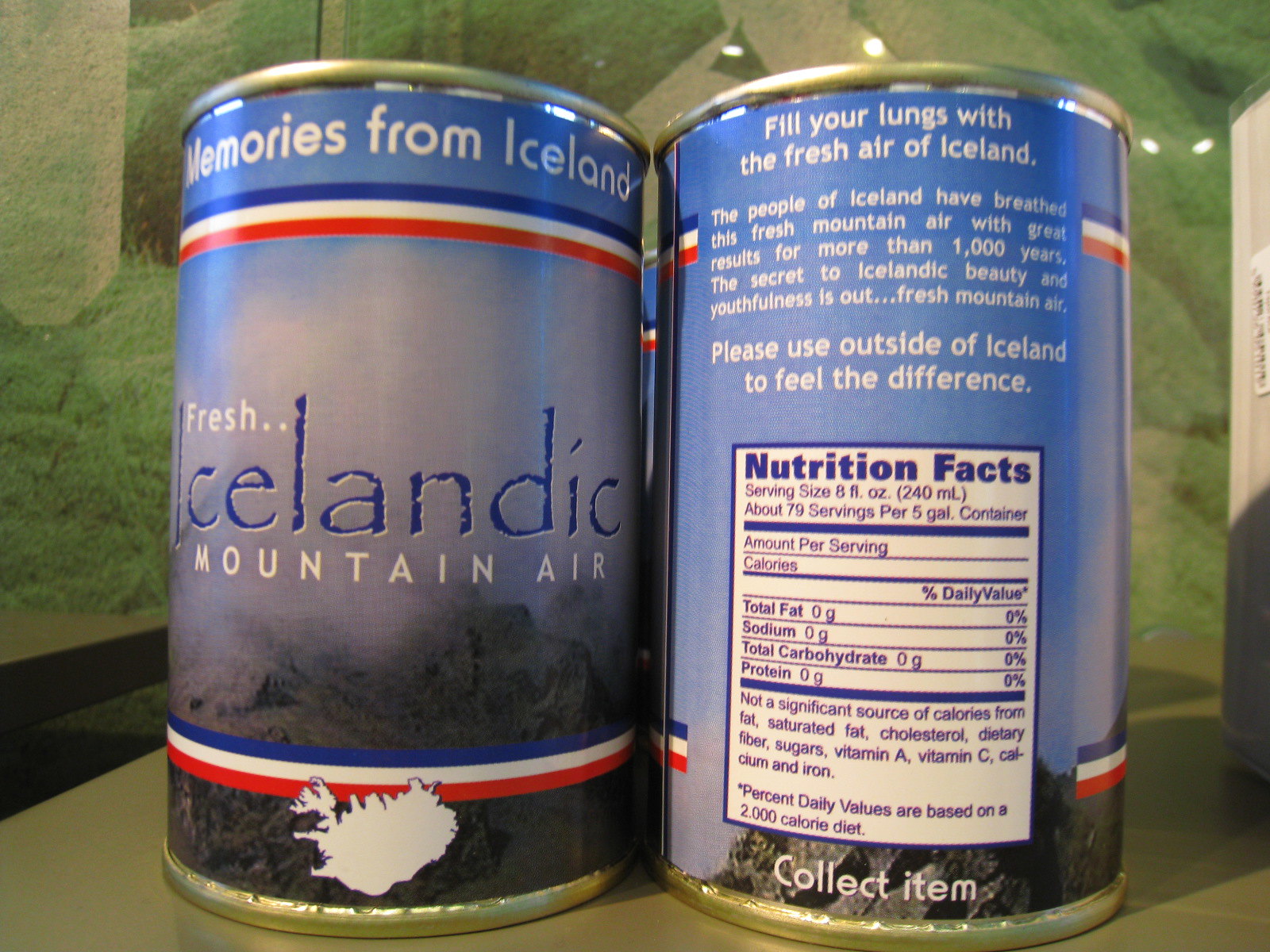This image depicts two novelty joke cans of "Fresh Icelandic Mountain Air" positioned side by side on a pale green table against a pale green background. The can on the left shows the front label, which features red, white, and blue stripes, a small outline map of Iceland, and the text "Memories from Iceland" at the top, followed by "Fresh Icelandic Mountain Air." The can on the right displays the back of the label, predominantly blue, with the text, "Fill your lungs with the fresh air of Iceland. The people of Iceland have breathed this fresh mountain air with great results for more than a thousand years. The secret to Icelandic beauty and youthfulness is out: fresh mountain air. Please use outside of Iceland to feel the difference," along with nutritional facts and "Collect item" at the bottom. The cans evoke the appearance of typical consumer goods, adding to their humorous appeal.